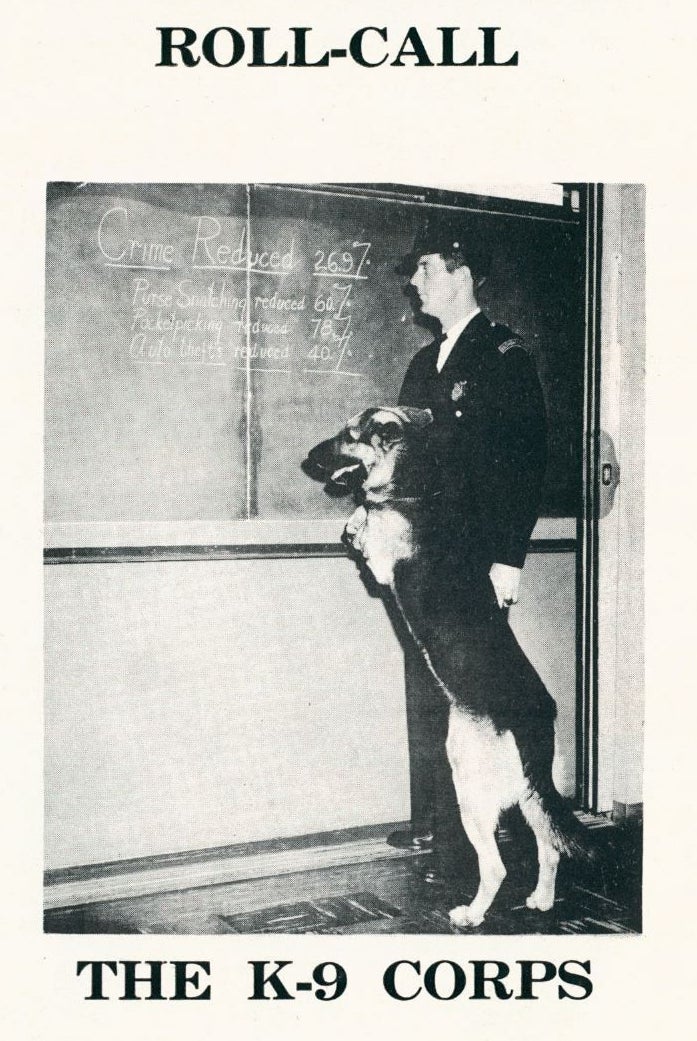This black-and-white photograph, likely from the early 1900s, captures a poignant moment during a 'Roll Call' session. The image prominently displays a police officer in uniform standing in profile, closely observing a chalkboard alongside his canine companion. The dog, also in focus, stands on its hind legs, seeming to read the chalkboard. The chalkboard features significant crime reduction statistics: "Crime Reduced 26.9%, Purse Snatching Reduced 60%, Pickpocketing Reduced 78%, Auto Thefts Reduced 40%." The setting resembles a classroom with a tiled floor, underscoring a sense of training or briefing. Above the scene, in bold text, 'Roll Call' is written, while at the bottom, the text 'The Canine Corps' signifies the specialized unit these two belong to.